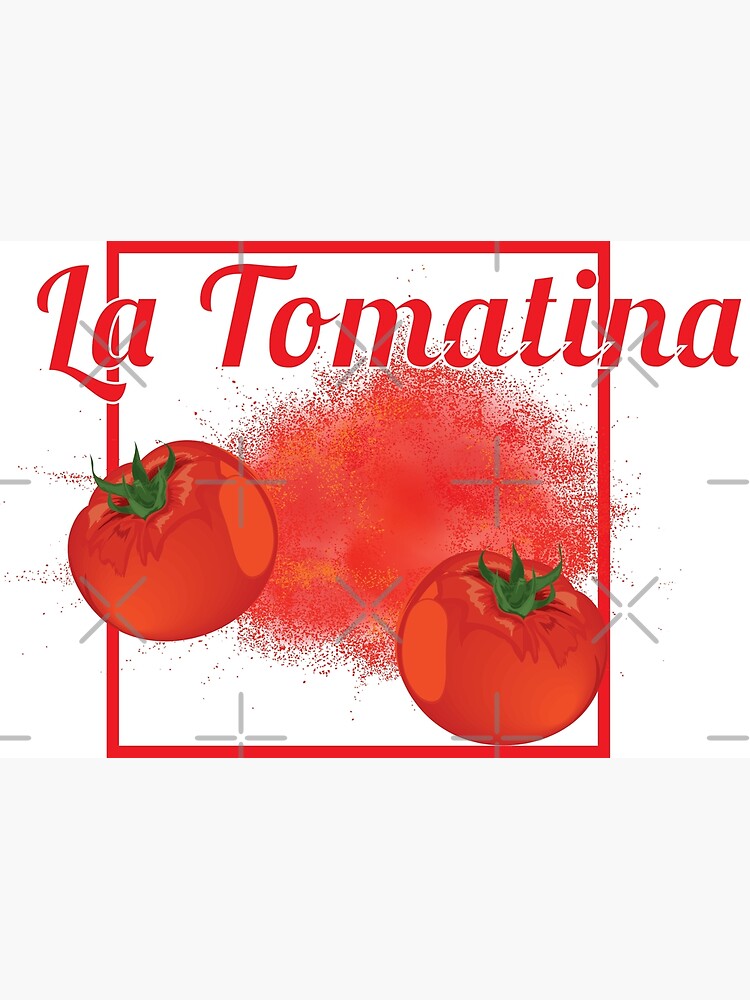The image appears to be a graphic poster, possibly for a restaurant, prominently featuring the text "La Tomatina" in cursive red letters at the top. Below this, a vivid red square frames two realistically-drawn round tomatoes with green stems, one positioned partly outside the frame. The background is predominantly white, accented with a subtle red splatter behind the tomatoes, giving the impression of spray paint. Additionally, the faint gray lines, reminiscent of a fragmented graph paper pattern, intersect at various points in the backdrop, adding texture without overwhelming the design. The overall aesthetic is clean and minimalistic, giving it a modern, brand-like feel.